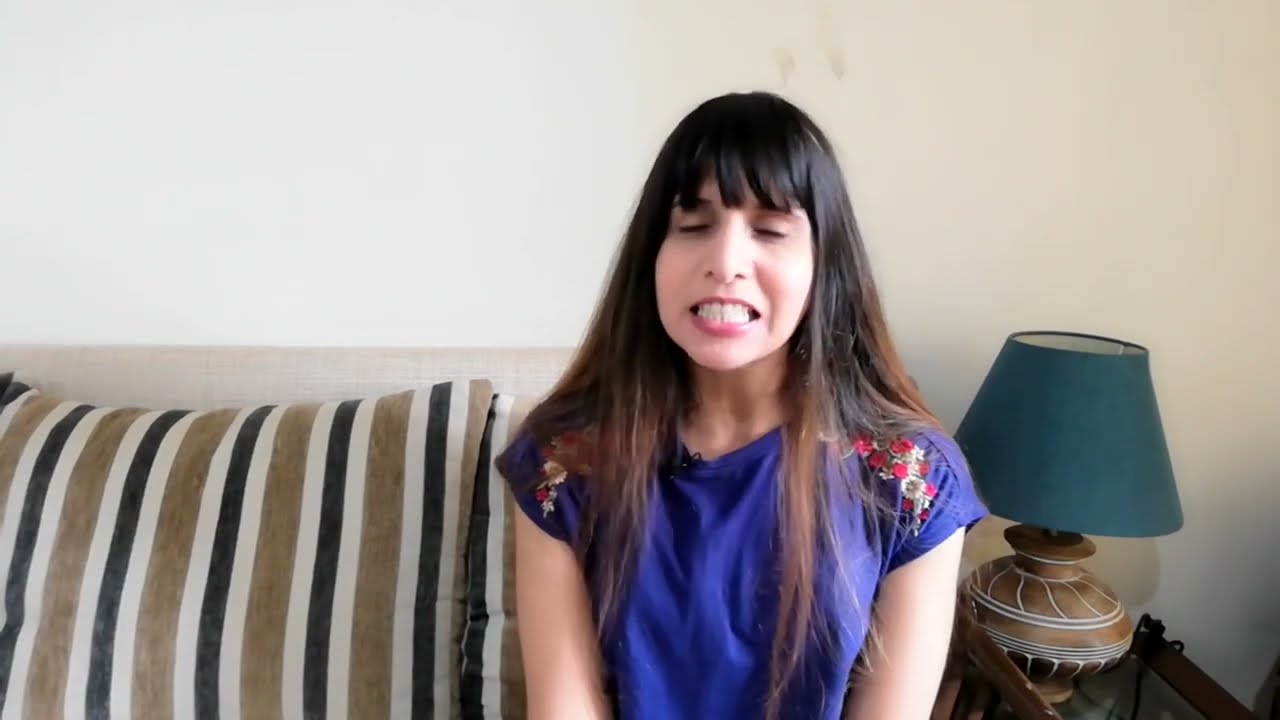In the photograph, a light-skinned woman with darker brown hair extending beyond her shoulders is seated on a beige striped couch. She is captured with her eyes closed and mouth open, gritting her teeth in what appears to be a spontaneous, unprepared moment. The expression on her face suggests a mixture of disgust and surprise. She's dressed in a purple short-sleeved blouse that features flowery patches on either shoulder in the front. Behind her, the couch is adorned with pillows with green, gold, and white stripes. To her right stands a lamp with a green lampshade and a brown base. The backdrop is white walls, adding a minimalist touch to the indoor setting. The photo, inadvertently amusing, seems to catch her off guard, making it a candid and genuine capture of a fleeting, unposed moment.